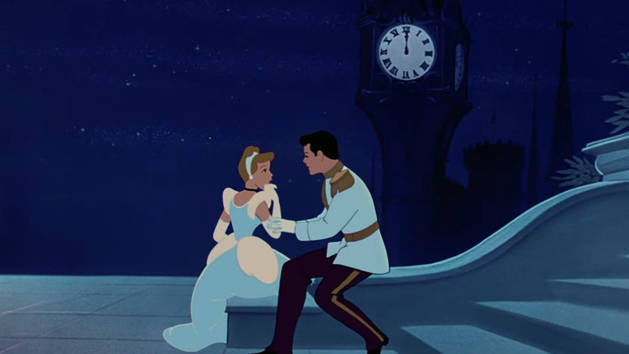In this still from the 1950s Disney movie "Cinderella," Cinderella is depicted wearing her iconic light blue dress with elegant white shoulders and gloves, complemented by a light blue headband and a striking black necklace. She sits on the steps with a surprised look on her face, speaking to Prince Charming, who is dressed in a light blue military jacket adorned with tassels and paired with black pants. His black hair contrasts sharply against his attire as he attentively listens to her, holding her right hand with both of his. Behind them, a grand clock tower is striking midnight, with additional towers silhouetted against the night sky. This scene encapsulates the magical moment when the spell is about to break, adding a dramatic and enchanting ambiance.